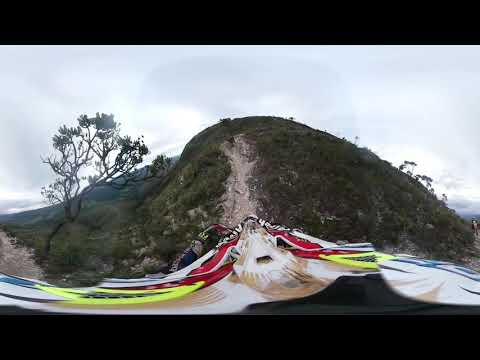In the foreground of the image, an all-terrain vehicle with a colorful hood, featuring red, yellow, and dark blue, is seen navigating a steep dirt trail that ascends a large hill. The GoPro camera captures the scene from behind the vehicle's hood, emphasizing the rugged terrain. The hill, steep and potentially part of a mountainous region, is bordered by grass, weeds, and small shrubs on either side of the trail. To the left of the hill, a sparse tree with branches that appear to be dying stands prominently in front of the hill. The sky overhead is gray and heavily clouded, suggesting an overcast day. The image also hints at a peculiar, possibly distorted object or figure at the front of the scene, which some might interpret as resembling a puffer fish with a beard or a person in a red bonnet with yellow accents. The overall setting evokes a rugged, natural landscape with a touch of whimsy in its unusual foreground.